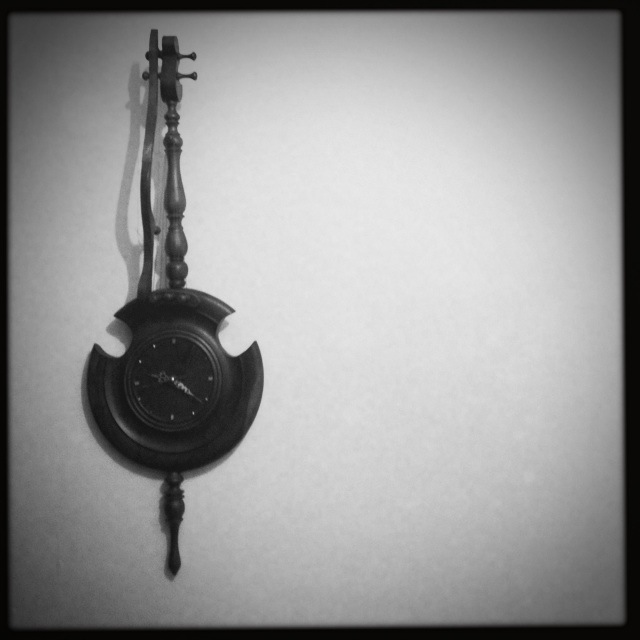This black-and-white grayscale image captures a stylized wall clock, which appears to be carved from dark wood. The clock features a unique design, reminiscent of a musical instrument. At the top, a rod resembling the neck of a guitar extends upwards, showcasing intricate carvings. Another wooden stick, seemingly conjoined at the top with strings running down its length, adds to the musical illusion.

The circular clock face is minimalist, adorned with just small dots in place of numbers. Two stylized, likely metal hands mark the time. Intriguingly, the circular body of the clock has two rounded indentations on either side, adding to its distinctive appearance. Extending from the bottom is another ornately carved wooden rod, further emphasizing the artistic craftsmanship of this eye-catching timepiece.